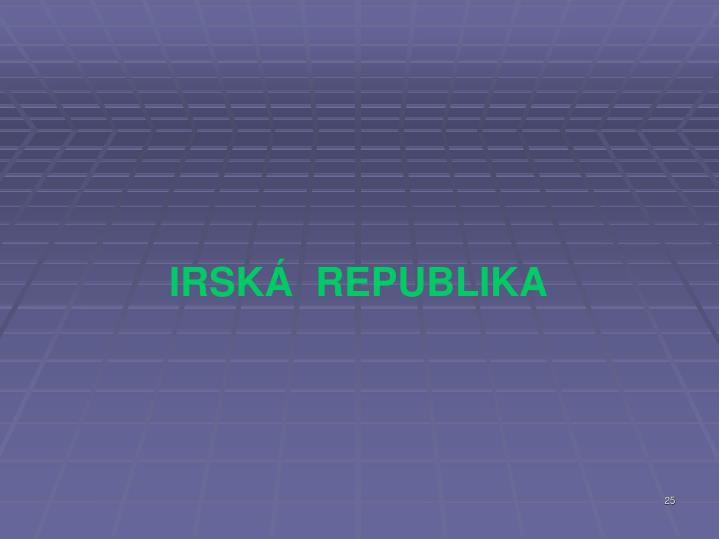The image appears to be a PowerPoint slide with a dark grayish-blue, checkerboard-patterned background that has a 3D effect, giving it the illusion of depth. The entire background, composed of small squares, has a subtle purple hue. In the exact center of the slide, there's green, capitalized text reading "IRSKA REPUBLIKA," with an accent on the "A" in "IRSKA." This text is prominently featured as the only wording on the slide. Additionally, in the bottom right corner, the number "25" is displayed in white.